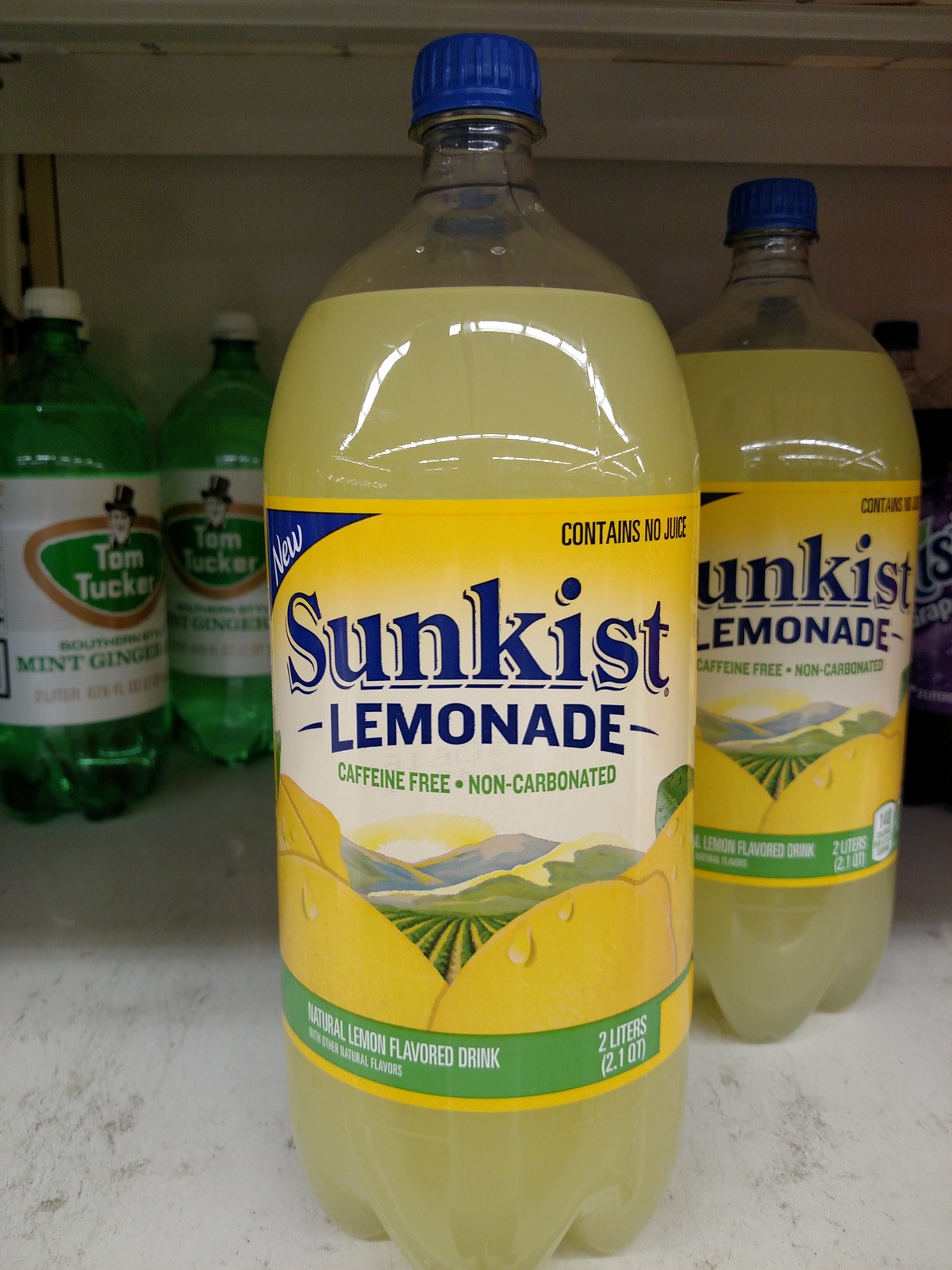The photograph captures a store shelf with a variety of beverages. The central focus is on 2-liter plastic bottles of Sunkist Lemonade. Prominently, one bottle in the middle displays a distinctive yellow label with blue lettering. The label features the signature "Sunkist" in navy blue, followed by "Lemonade" in a unique font where the letters "L" and "E" are capitalized and slightly larger. The top left corner of the label highlights "New" in white cursive, while the top right corner states "Contains No Juice" in navy blue capital letters. Below "Lemonade," it reads "Caffeine Free Non-Carbonated" in a lime green font. The label also includes an illustration of a picturesque scene: a blazing white sun over distant green mountains and meadows, with oversized lemons in the foreground, giving the impression of "lemon mountains."

At the base of the label, a lime green band features the text "Natural Lemon-Flavored Drink" in white capital letters, along with smaller text stating, "With Other Natural Flavors." The total volume of the bottle, 2 liters, is displayed on the far right of the lime green band.

Adjacent to the centerpiece, another bottle of Sunkist Lemonade is slightly behind it, partially visible. Surrounding these are several bottles of Tom Tucker Mint Ginger Ale, easily recognizable by their green labels, white caps, and a distinctive design featuring a black top-hatted man with a white beard. This ginger ale's label includes the name "Tom Tucker" in white, surrounded by a green band and a red stripe detail.

The entire arrangement is set on a simple white store shelf, creating a clean and organized presentation of the beverages.